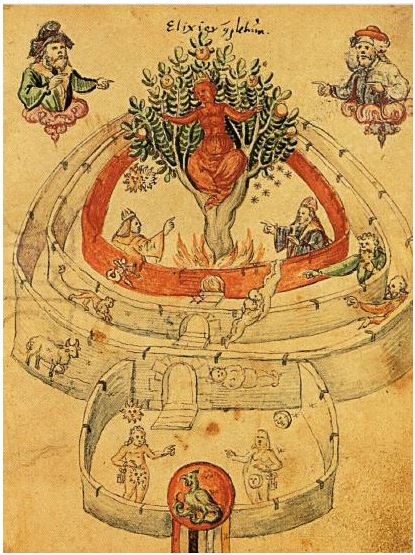This detailed alchemical illustration is drawn on an old, faded yellow parchment, marred by brown spots and stains. The image's upper left corner features a man in green and yellow robes with a gray hat, pointing towards the illustration's center, while on the right side, an older man with white hair, donned in white robes and a red hat, also gestures towards the center. The scene unfolds below into a labyrinthine courtyard populated with a plethora of figures, including kings, ghostly spirits, sheep, lions, and satyr-like creatures, arranged within various levels of the maze.

Central to this intricate tableau is a red wall encircling a significant motif: a burning tree adorned with green leaves and orange fruit. Nestled amid the flames is a striking blood-red female figure, wearing a tiara, her arms outstretched. The tree emanates a sense of alchemical transformation, with kings below pointing upward towards it. The background tone of the parchment is tan or brownish, adding to its aged appearance. Additionally, annotated at the top in handwritten pen is the enigmatic word "elixir," possibly "X-E-L-I-X-I-E-R," hinting at the mystical nature of the illustration.

Complementing the scene are Scandinavian gnome-like figures in the top corners and various animals and cherubs scattered throughout the courtyards. The composition is rich in symbolism, with figures interacting in seemingly dialogical poses and others girded in moments of contemplation or conflict, encapsulating a visual journey through esoteric allegory.